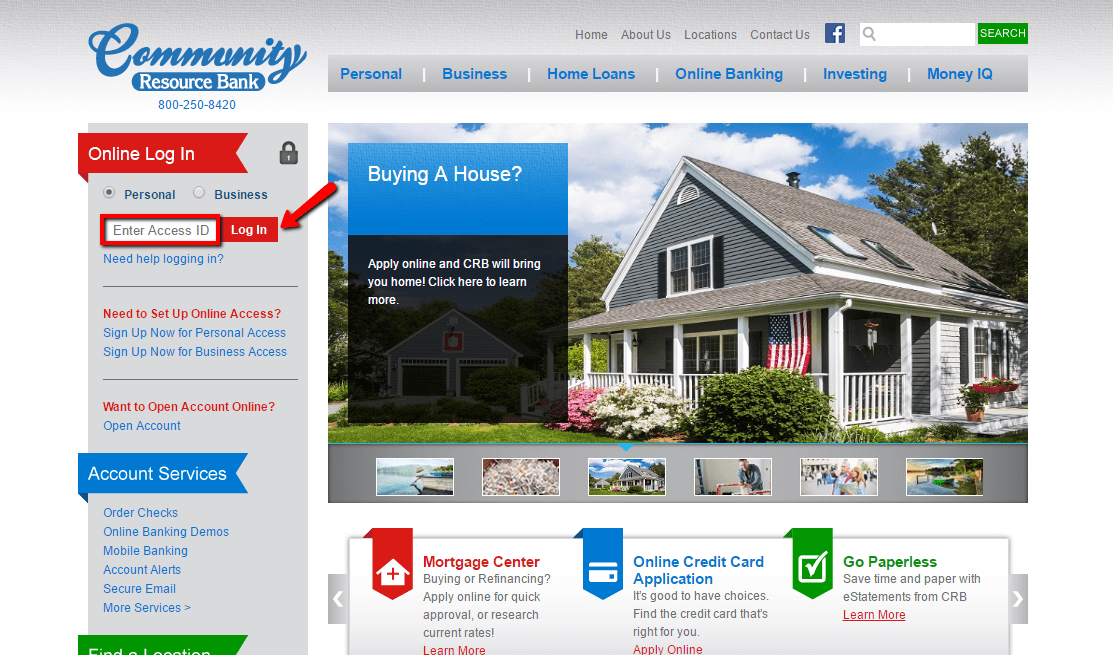This image is a detailed screenshot of a webpage from the Community Resource Bank. The design is a horizontal landscape with a gradient background that transitions from gray at the top to white at the bottom. 

In the upper left corner, the text "Community Resource Bank" is prominently displayed alongside a contact number, 800-250-8420. Spanning the top of the page, there's a navigation bar featuring various menu options: Personal, Business, Home Loans, Online Banking, Investing, and MoneyIQ.

On the left side of the page, there's a vertical gray box labeled "Online Login" with further prompts. It instructs users to enter their Access ID into a designated field and features a prominent red "Login" button. Below this, support prompts are listed: "Hello, Need Help Logging In?", followed by options for setting up online access, including "Sign up now for personal access" and "Sign up now for business access." Another prompt encourages prospective users to "Open an account online."

Further down, a blue banner titled "Account Services" lists additional services such as Order Checks, Online Banking Demos, Mobile Banking, Account Alerts, Secure Email, and More Services.

Occupying the right side of the page is a large image of a house with white siding and a gray roof, set against a spacious green lawn. Next to this image, a blue box contains the text "Buying a House" in white, and directly below, a black box with white text reads "Apply Online and CRB will bring you home. Click here to learn more."

Underneath the house image, there are smaller images, though these are not described in detail.

This comprehensive webpage offers various banking services and navigational aids, creating a user-friendly experience for customers of the Community Resource Bank.